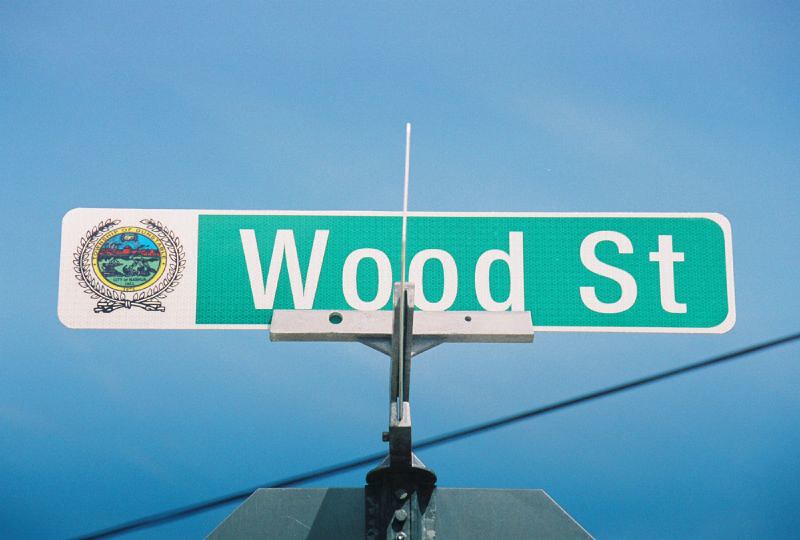This outdoor photo showcases a green banner-type street sign that reads "Wood Street" in white print. To the left side of the sign, there's a circular state or city seal on a white background, with a yellow border and a decorative wreath at the bottom, tied with a bow. Inside the seal, there are intricate elements in green, blue, and red script, though the text is illegible. The sign itself is unusually mounted on a structure resembling a music stand, with a single pole and a bar supporting it. The contraption appears to be makeshift, precariously attached to a black, metal object of indeterminate function. A power line is visible behind the sign, suggesting the photo might be taken from an unconventional angle, adding to the impression that the sign is temporarily affixed in an atypical manner.